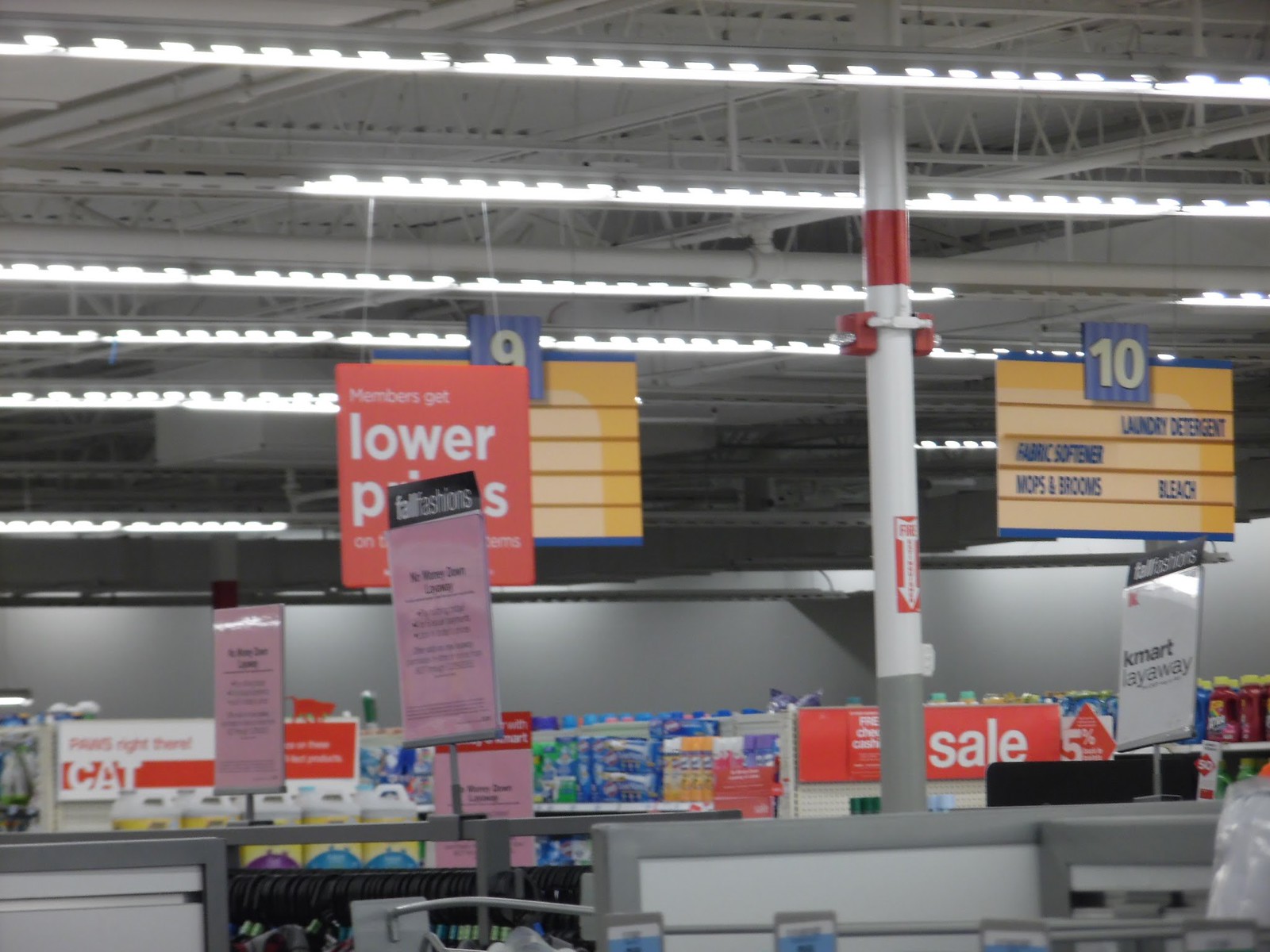This photograph captures the interior of a Kmart store, highlighting a variety of overhead aisle signs and product displays. Prominently, there's a "Kmart Layaway" sign, establishing the store's identity. Overhead, other signs designate the aisles: aisle 9 and aisle 10, the latter detailing products like laundry detergent, fabric softener, mops and brooms, and bleach on a yellow sign. A red sign stating "Members get lower prices" partially obscures the aisle 9 sign. The photograph, though out of focus, hints at shelves stocked with various household items, including cleaning solutions and spray cans. The store's open layout is evident with its exposed utilities and gray ceiling, illuminated by fluorescent white lights. The walls and shelves are also gray, adding to the industrial aesthetic. Additional signs for seasonal promotions like "Fall Fashions, Lower Prices" are visible, contributing to the retail atmosphere.